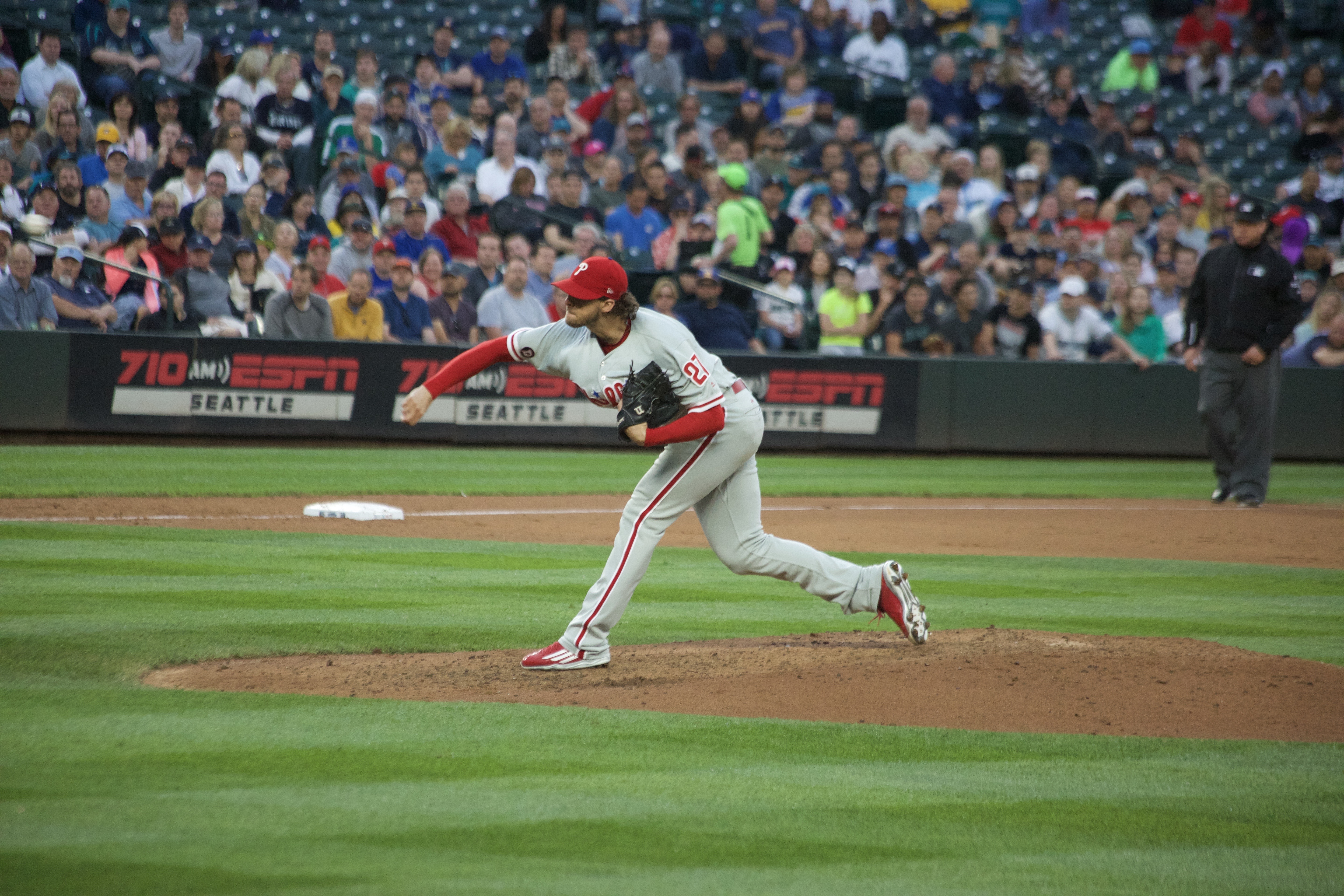The image depicts a Major League Baseball game featuring a pitcher from the Philadelphia Phillies, identified by his last name "Nola," during an action-packed moment on the mound. Nola, wearing a gray uniform with red numbers and detailing, is captured mid-pitch, with his right arm fully extended and his left hand sporting a dark brown glove. His attire includes a red long-sleeve shirt under the jersey, contributing to the vibrant contrast with his gray uniform, and he is donning a red cap with a white "P" emblem. His left leg firmly plants on the ground, while his right leg is slightly raised, showing dynamic motion. In the background, an official dressed in a black jacket, gray pants, and a black hat can be seen near third base, overseeing the game. The stadium's barricade displays an advertisement for "710 AM ESPN Seattle," adding context to the setting, while a lively crowd fills the stands, attentively watching the unfolding action.